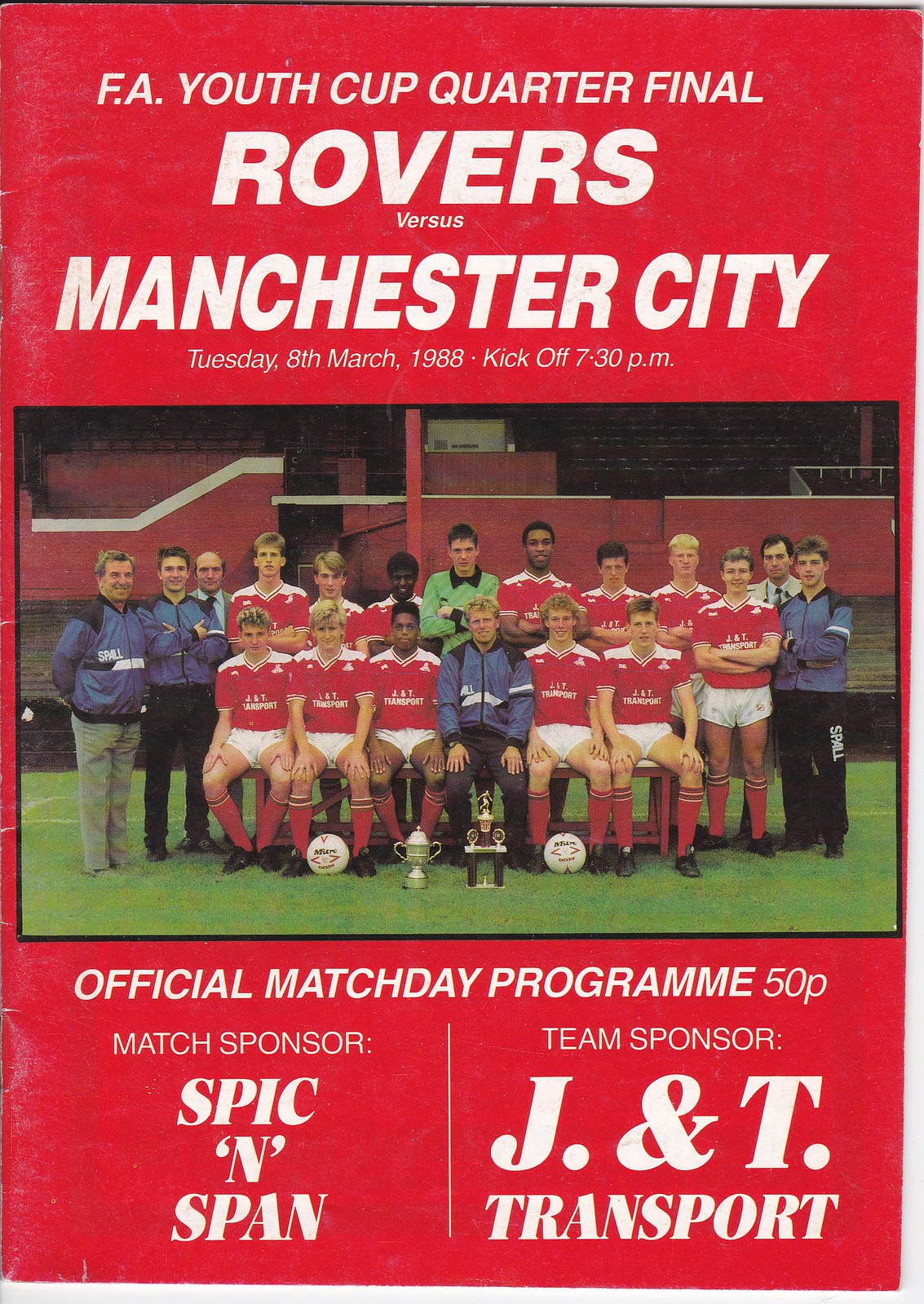This poster is for a soccer match, prominently displaying a photo of the players and coaches in the center. The players are dressed in red and white jersey tops, white shorts, knee-high red socks, and black shoes. In the photo, some players are seated while others stand, with coaches in blue jackets and varied pants. A standout individual in a green top is also visible. In front of the group, there are two soccer balls and two trophies. The backdrop features a soccer field and a stadium. The cover's bright red background contrasts with the bold white text that reads, "F.A. Youth Cup Quarter Final, Rovers vs. Manchester City," scheduled for Tuesday, 8th March 1988, with a kickoff at 7.30 PM. Additional text at the bottom announces, "Official Match Day Program, 50P," with sponsorship details: "Match Sponsor: Spick and Span" and "Team Sponsor: J&T Transport." The word "program" is notably spelled with two "m"s and an "e."